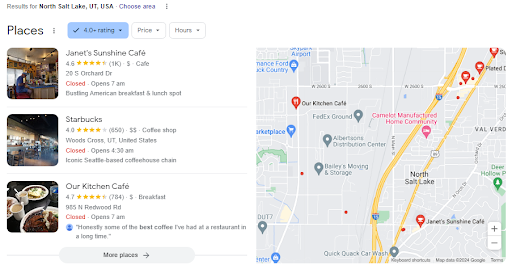Here is a revised and descriptive caption for the image:

---

The image showcases a digital search result screen, likely from a computer or mobile device, with results for "North Salt Lake, Utah, USA." At the top, there is an option labeled "Choose Area." Below this, there are categorized listings under "Places," filtered by establishments with a 4.0+ rating, highlighted in a blue box. Adjacent to it are filters for "Price" and "Hours." 

The first listing shows a bustling American breakfast and lunch spot named "Janet's Sunshine Cafe" with a rating of 4.6 stars. Despite being currently closed, its address is visible. Below it, the second listing features the iconic Seattle-based coffeehouse chain "Starbucks," with a 4.0-star rating. This location is noted to open at 4:30 a.m. The third and final visible listing is "Our Kitchen," showing an inviting image of plates filled with food on a table, rated highly at 4.7 stars. This establishment opens at 7:00 a.m. 

The entire right side of the screen is dedicated to a detailed map highlighting the locations of these restaurants with pins, allowing users to locate them easily and explore others in the vicinity.

---

This caption provides a comprehensive and detailed description of the image contents.